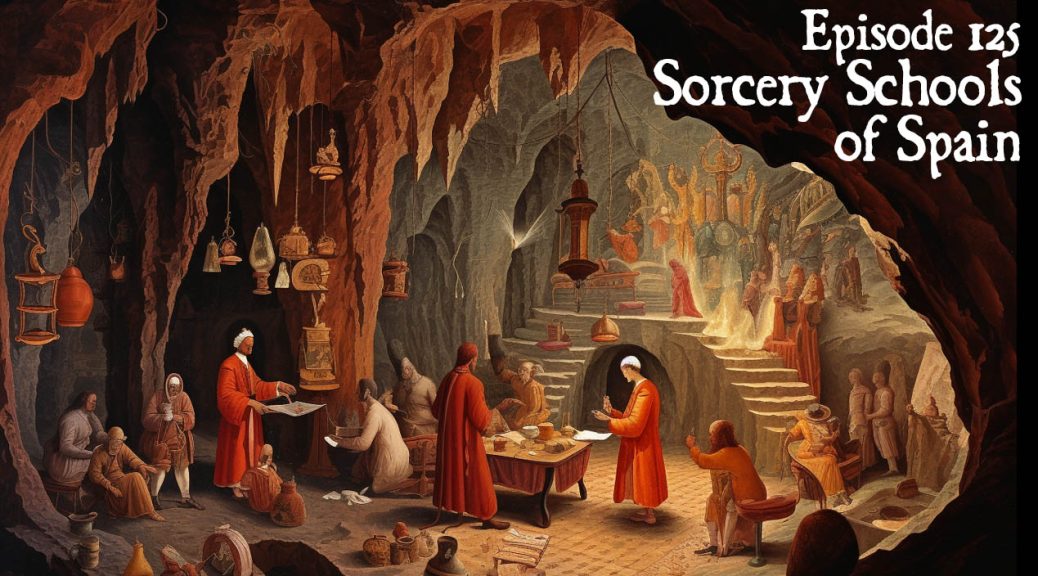The rectangular thumbnail, possibly for a YouTube video titled "Episode 125, Sorcery Schools of Spain," features a colorful illustration reminiscent of work done in colored pencils or oil pastels. The image presents a cavernous underground school or temple, adorned with stalactites hanging nearly to the ground and various medium-sized vessels, including pots, a deer head with hanging baskets, and lanterns suspended from the ceiling. Numerous people, dressed in red-orange and beige robes, some with white or red caps, populate the scene, engaging in various activities around several tables with cups and other objects. Central to the illustration is a table surrounded by these robed figures. In the background, a platform with a staircase on each side leads up to an elaborate altar, which features a golden pillar, decorative ornamentation, a chest, and multiple idols, creating an impression of an ancient and mystical culture within the cave's sandy floor setting.